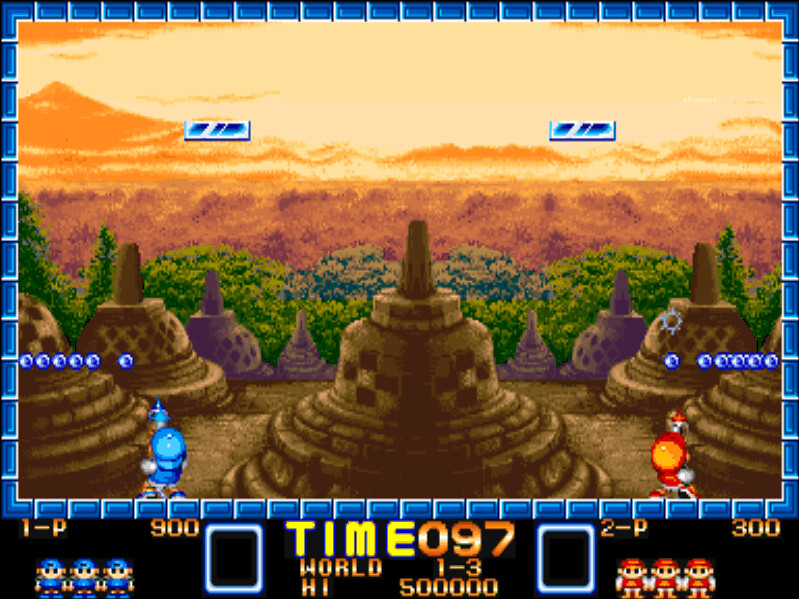This image depicts a scene from a classic, pixelated video game reminiscent of the Atari 2600 era. On the left side of the screen, a character dressed in blue stands poised, while on the right, another character adorned in orange is present. The pixelated graphics evoke nostalgia for old-school gaming enthusiasts. Each character has a row of six blue dots above their heads, with a unique spacing that separates a single dot from the group of five.

At the top section of the frame, two small blue bars are visible. The background features an orange-tinted sky, accompanied by pixelated green trees and various building-like structures interspersed throughout. The score for Player 1 is displayed as 900, while Player 2 has a score of 300. The timer shows 97 seconds remaining, indicating the game is set in World 1-3. The high score noted in the game is an impressive 500,000 points.